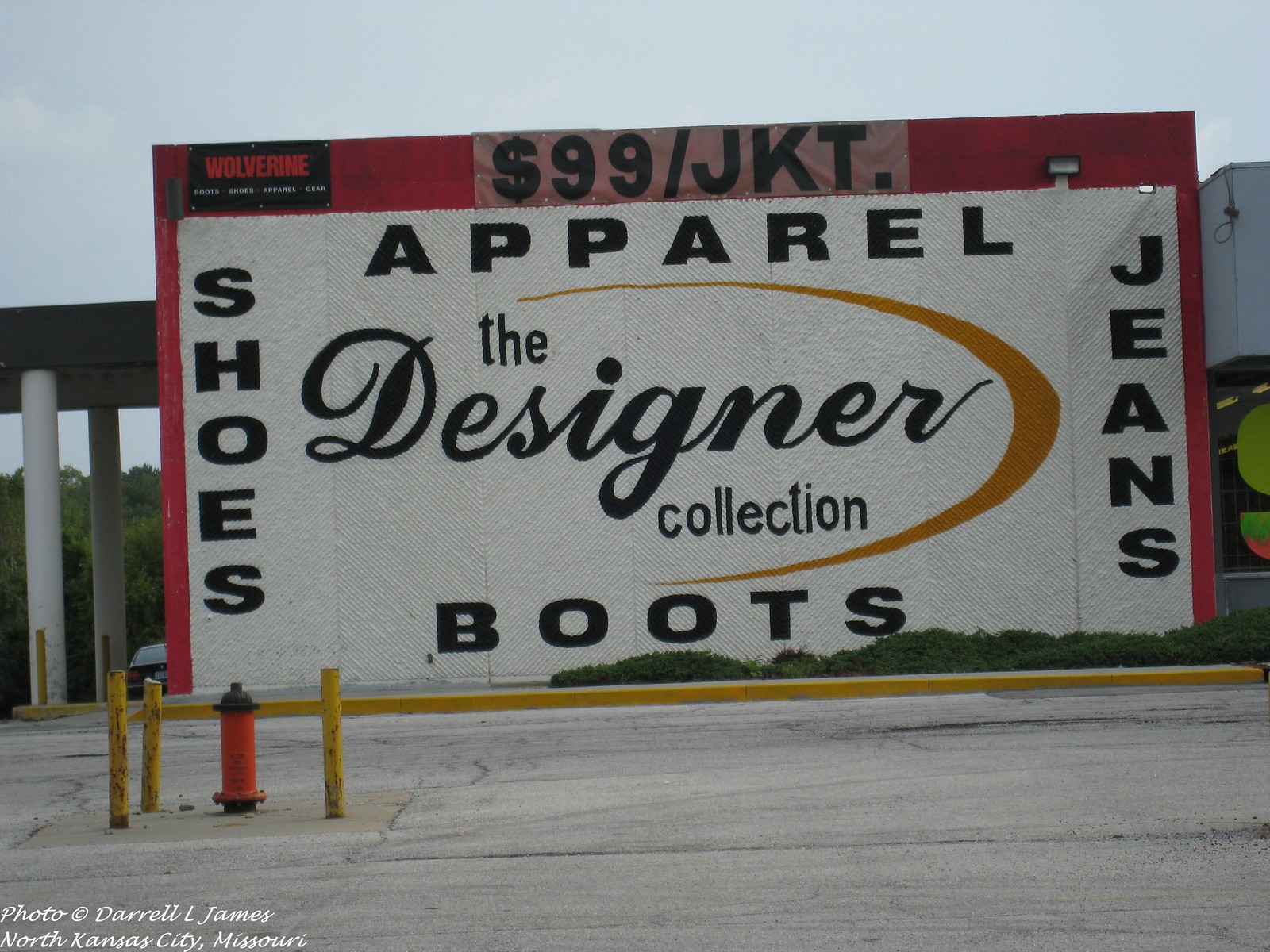This image depicts a very large rectangular business sign, approximately 20 to 30 feet high and 40 feet wide, prominently displayed against what appears to be a bridge or possibly the wall of a building. The sign features a red border with varying thickness, thinner on the sides and slightly wider on the top. At the top of the sign, large black letters read "$99-JKT," indicating a price for jackets. 

In the center of the sign, the phrase "Apparel, The Designer Collection, Boots" is displayed, with "Designer" elegantly written in cursive. Surrounding "The Designer Collection," is an orange, almost boomerang-shaped logo, possibly representing the brand's icon.

Additionally, the words "Shoes" and "Jeans" are vertically oriented on the sides of the sign, with "Shoes" on the left and "Jeans" on the right. To the left of the sign, three yellow posts partially enclose what looks like an orange fire hydrant with a black top, though it's not entirely clear. 

The entire scene is set against an empty parking lot with two white columns supporting an awning or walkway structure to the left of the sign, enhancing the industrial ambiance of the location.